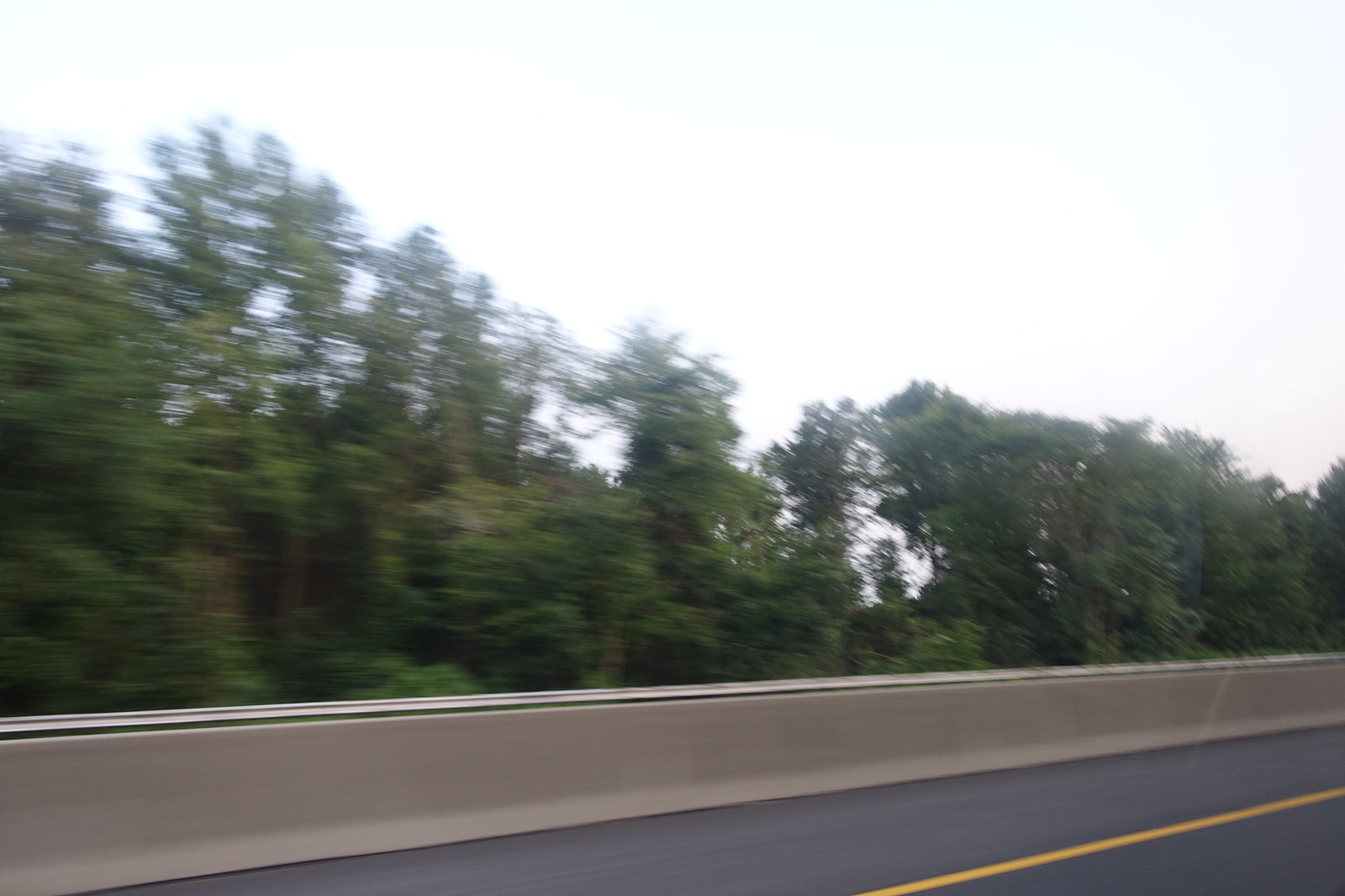This photograph captures a scenic roadside view, where the bottom right corner and edge reveal an asphalt road marked with a diagonal orange line. Dominating the foreground is a gray-white concrete Jersey barrier, which adds a man-made contrast to the natural elements in the background. Just behind the barrier, a line of trees stretches horizontally, their tops softly out of focus, adding a dreamy quality to the greenery. Above the trees, a voluminous white puffy cloud creates a striking presence against the very light blue sky. A subtle detail emerges on top of the Jersey barrier, resembling a pipe made of silver metal, adding an interesting industrial touch to the overall composition.